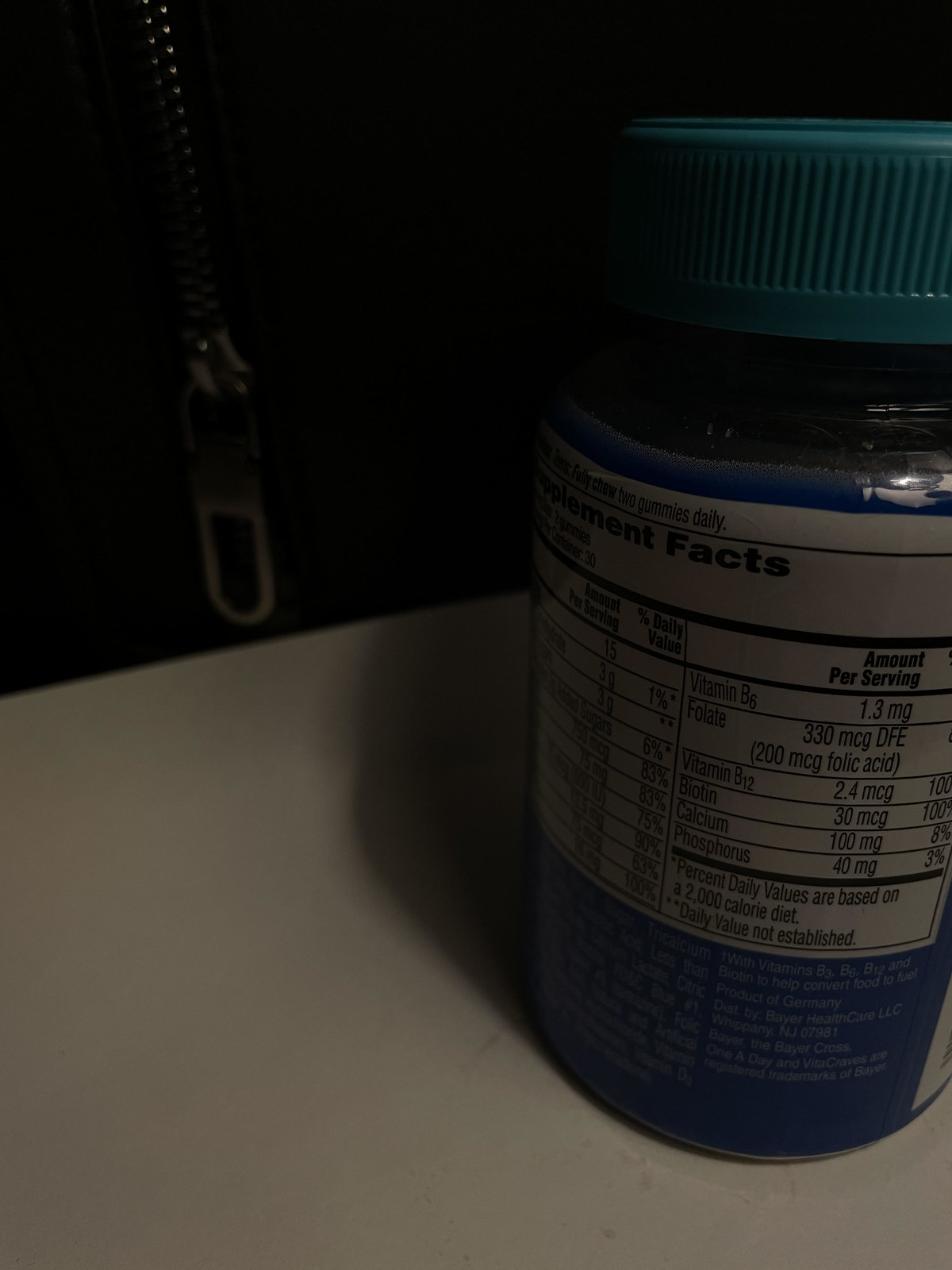This dimly lit color photograph features a scene in which a jar is prominently placed on a light gray counter to the right. The jar, though somewhat shadowed and not entirely clear, sports an aquamarine blue lid. The jar's label displays nutritional facts, though the text is unreadable due to the small print and poor lighting. Below the nutritional label, the bottom part of the bottle's label appears, in a royal blue background with elusive silver print. In the upper left corner of the image, a zipper from what seems to be a jacket is partially visible. The zipper's teeth can be seen at the top, with the zipper handle or loop near the counter's edge. The overall ambiance of the image is heavily subdued due to the very dim lighting conditions.